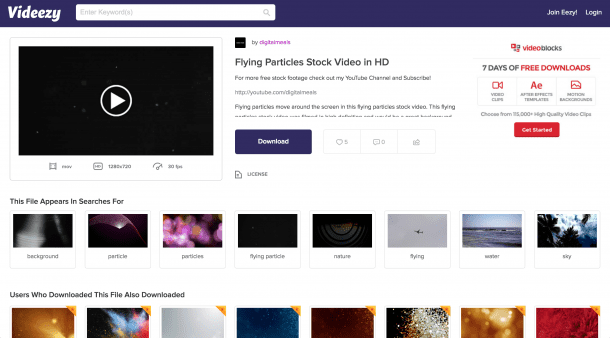A screen capture from the Vidizi website showcases its interface and features. The top section includes a blue navigation bar with the Vidizi logo in white, accompanied by a white search bar and options to "Join Today" or "Log In." Prominently displayed is a black video screen with a play button icon, labeled "Flying Particles Stock Video in High Definition," available for download.

Beneath the video screen, the file is tagged with search terms such as "background," "particles," "nature," "flying," "water," and "sky." A section titled "Users who downloaded this file also downloaded" presents thumbnails of additional stock footage options, featuring a variety of colors and themes like gold, colorful patterns, neutral tones, stars, twinkling lights, and close-ups of red roses.

On the top right corner, a promotional banner for VideoBlocks offers a seven-day trial with access to 115,000 high-quality video clips and motion backgrounds. Users are prompted to get started by clicking a red button to begin their free downloads.